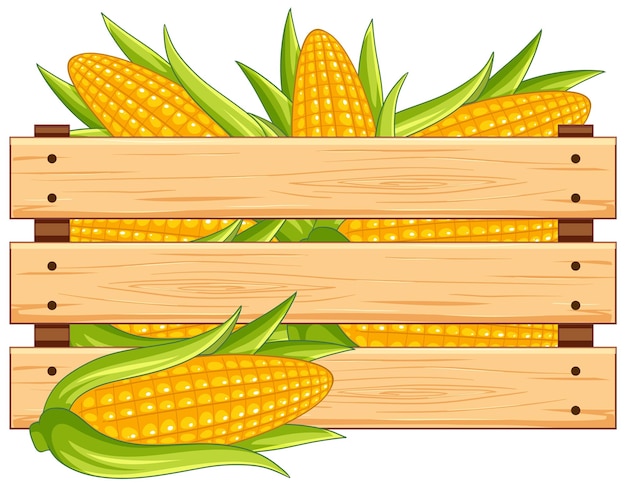In this detailed digital illustration, a wooden crate filled to the brim with fresh corn cobs occupies the foreground. The crate, constructed of pale, light brown wood, comprises three horizontal planks fastened with nails, creating slight gaps through which the vibrant yellow corn kernels and lush green husks peek. The meticulously arranged corn fills every centimeter of the crate, giving an impression of abundance. Notably, one corn cob has tumbled out, lying prominently in front of the crate, its husk still intact and the golden kernels glowing. Set against a plain white gradient background that provides contrast and highlights the bright colors of the corn, this image captures the rustic charm and fresh appeal of harvested corn ready to be eaten or sold.